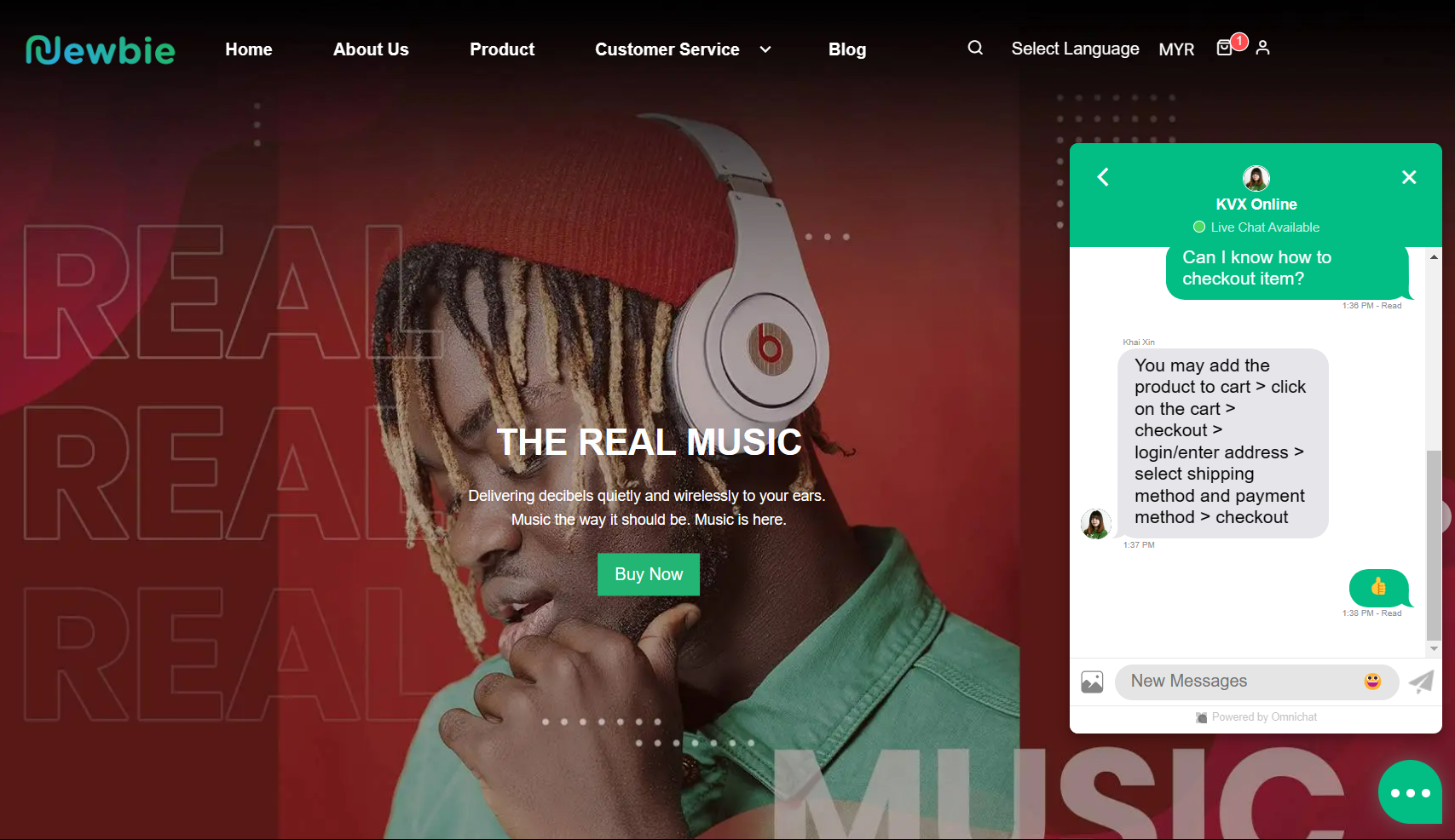Screenshot Description: Desktop App Interface

This screenshot showcases the interface of a desktop application. The top left corner prominently displays the word "Newbie" in a font comprised of a blend of blue and green letters. The exact font used is indeterminate. The app features a dynamic background that transitions between shades of black and red.

Adjacent to the company logo located in the same top left region, there is a navigation menu with the following options: Home, About Us, Product, Customer Service, and Blog. To the far right of these options, a magnifying glass icon is present, which likely serves as a language selection tool. Also in this area are a mail or notification icon marked with a red badge indicating '1', and a profile icon situated to its right.

Dominating the center of the screen is the tagline: "The Real Music, delivering decibels quietly and wirelessly to your ears. Music the way it should be. Music is a year. Buy now." Beneath this message, a prominent green "Buy Now" button invites user interaction.

To the right of the main content area, there is a bot messaging system labeled "KBX Online," indicating that live chat support is available. An informative green balloon message on the interface provides guidance on how to check out: "You may add the product to the cart, click on the cart, check out, log in, or enter the address, select shipping method and the payment method, and then check out." A prompt for initiating a new message is visible just below this information.

Overall, the interface is rich with navigational aids and interactive elements designed to facilitate an engaging user experience.